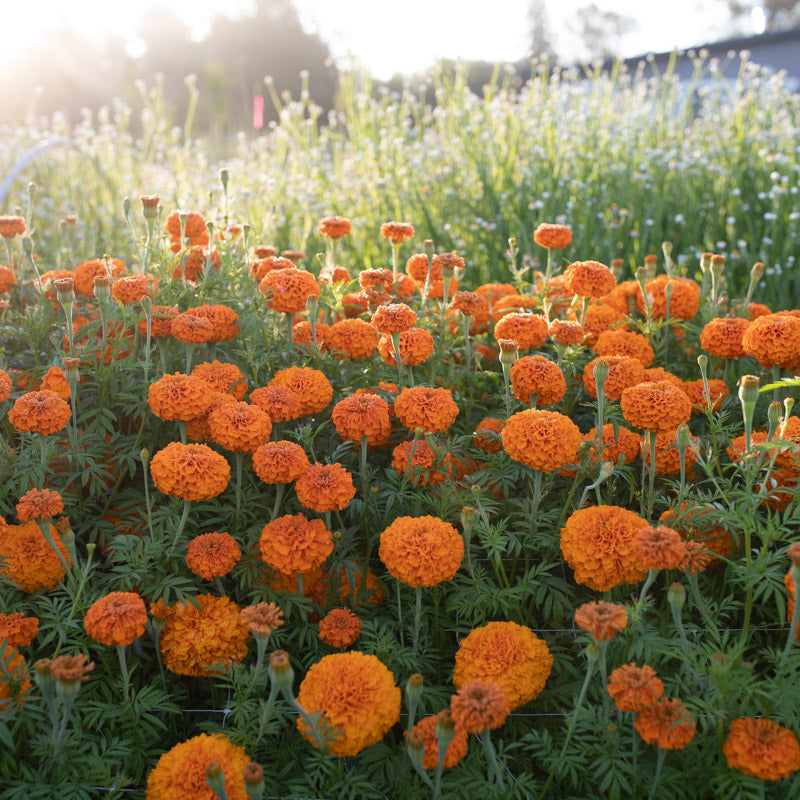This color photograph captures a vibrant field of orange flowers with round heads and long green stalks, filling the lower two-thirds of the image. These flowers display varying sizes and heights, some with a reddish tint at their centers. In the middle ground, tall plants with tiny white or blue-tinged flowers rise up, though slightly out of focus, adding depth to the scene. A tree line silhouetted against the bright sunlight is visible in the upper left, while on the right, the roof of a building with a white side and black gutter peeks out, framed by additional trees. The sky above is a bright white, emphasizing the sunny, luminous day captured in the photograph.